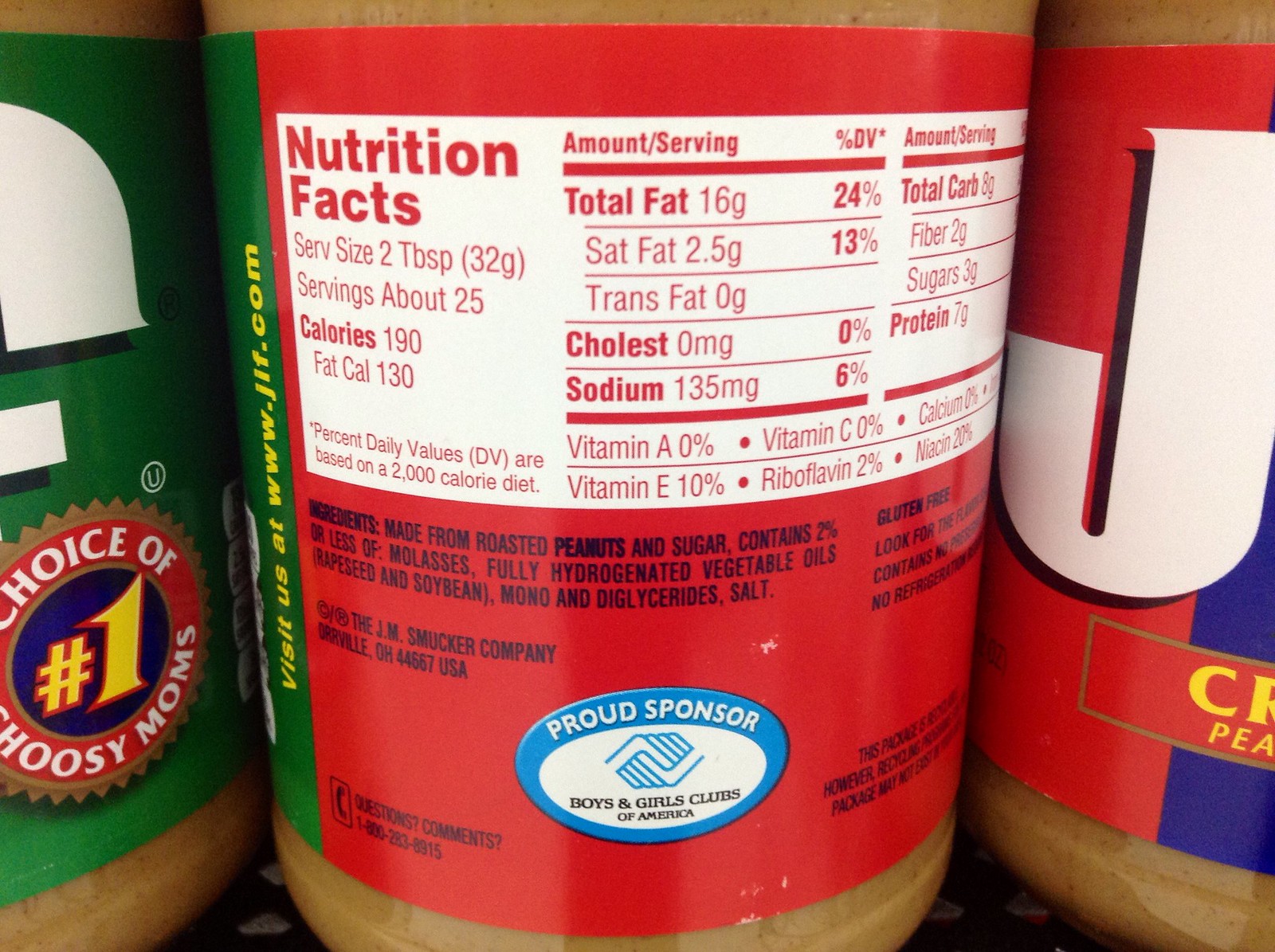This photograph captures the back of a Jif peanut butter jar, prominently displaying the Nutrition Facts label. The setting appears to be a market, evidenced by the presence of two additional Jif jars flanking the central one. The jar on the left is oriented forward, revealing the green segment of its label and a partial view of the 'F' in 'Jif', along with a slogan stating, "Number One Choice of Choosy Moms." The jar on the right is positioned to show the red portion of its label with a visible 'J'. Notably, at the bottom of the center jar's label, there is a small logo that proudly announces Jif as a sponsor of the Boys and Girls Clubs of America.